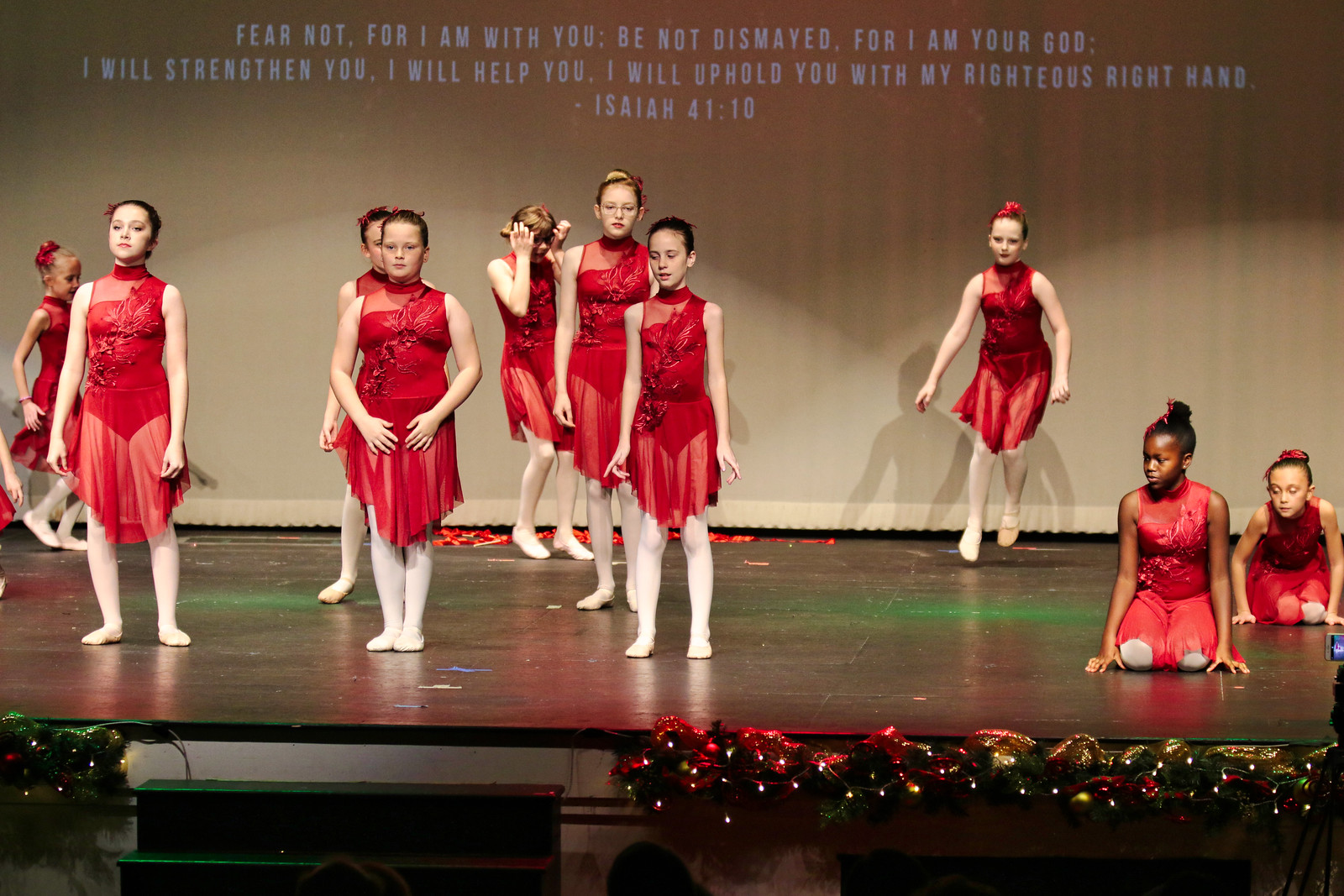This photograph captures a ballet performance on a black stage featuring a group of young girls, likely around 10 or 11 years old, dressed in red tutus with unevenly cut skirts that rise at the hips, paired with white leggings and ballet shoes. All dancers have their hair pulled back, and a few adorn bows, while one girl wears glasses. The performance has a diverse cast, including a Black girl and several white girls, with some standing, some posing, and two kneeling on the right. In the background, a beige curtain displays a quote in white text: "Fear not, for I am with you. Be not dismayed, for I am your God. I will strengthen you. I will help you. I will uphold you with my righteous right hand. Isaiah 41:10." The front of the stage is decorated with lighting and festive bow decorations, contributing to a Christmas-themed ambiance.